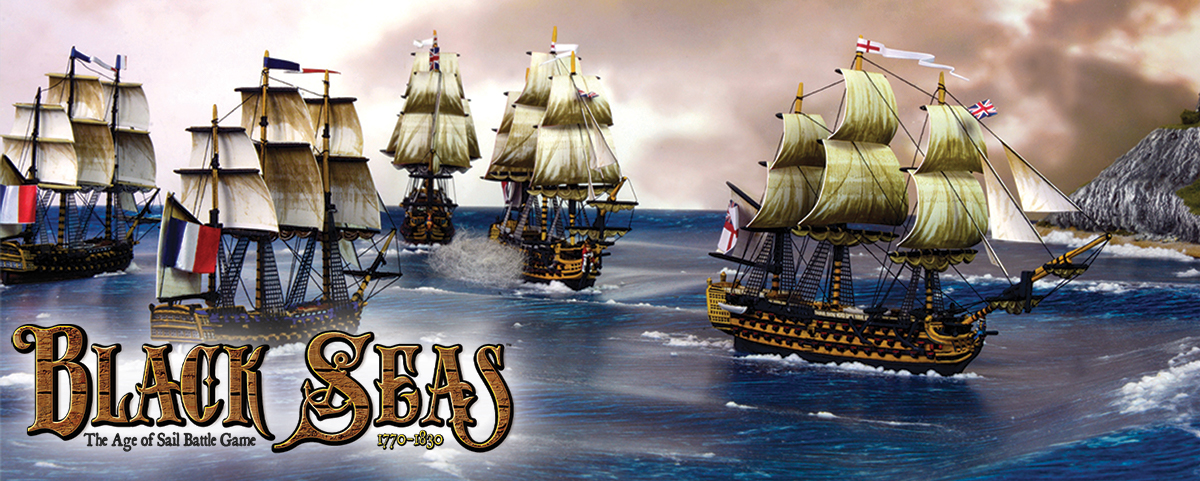This advertisement for the game "Black Seas: The Age of Sail Battle Game, 1770-1830," is set in a long rectangular format. The scene depicts five large sailboats navigating dark blue, wave-filled waters, with white bubbles forming on the surface. Each ship features multiple masts, some with six sails, and flies various flags from their tops. The leading vessel on the right is distinguishable by its white flag with a red cross and a British flag adorned with red, white, and blue lines. The hulls of the ships primarily display a dark brown base with yellow accents, giving them a weathered look. The background is dominated by stormy, dark gray clouds with streaks of orange light cutting through, suggesting an impending storm. The sky's overcast nature contributes to the dramatic and immersive atmosphere of the game. The game’s title, "Black Seas," is clearly displayed in the bottom left corner of the image, accompanied by the subtitle “The Age of Sail Battle Game, 1770-1830.”